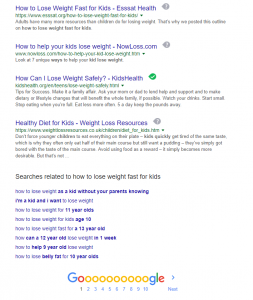The image depicts an old-school Google search results page. The nostalgic Google logo features multiple 'O's in the word "Google"; the first 'O' is red, and the remaining are yellow, reminiscent of older web interfaces. At the bottom of the image, there are page numbers ranging from one to ten, with a navigation option to proceed to the 'Next' page.

The upper part of the image shows a list of search results related to weight loss for children. However, many details are blurry, making it difficult to discern the full content. The first visible result is titled "How to Lose Weight Fast for Kids." The second result, attributed to nowloss.com, is "How to Help Your Kids Lose Weight." The third entry, marked with a green checkmark, reads "How Can I Lose Weight Safely - Kids Health." Another result is titled "Healthy Diet for Kids - Weight Loss Resources."

Below the search results, there is a "Searches related to 'how to lose weight fast for kids'" section. Some legible search queries include "How to lose weight as a kid without your parents knowing," "I'm a kid and I want to lose weight," "How to lose weight for 11 year olds," "How to lose weight for kids age 10," "How to lose weight fast for 12 year olds," "How can a 12 year old lose weight in one week," "How to help a 9 year old lose weight," and "How to lose belly fat for 10 year olds."

The context of these search queries is concerning, as it reflects the pressures faced by young children regarding weight and body image.